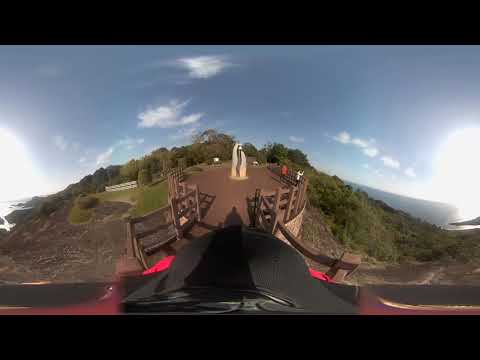The image appears to be an aerial shot, most likely taken from a drone, overlooking a scenic outdoor setting. The camera is positioned at an elevated angle, providing a broad perspective of the landscape. In the foreground, there's a grassy hill adorned with green shrubbery and a brown, circular walkway bordered by a brown fence. At the center of this circular space, a white concrete statue is visible, although the details of the statue are indistinct due to the distance. 

Behind this area, the image captures a dull blue sky dotted with white clouds, and some visual anomalies that look like two suns, likely due to a photographic filter. There are also a couple of white orbs on both sides of the sky, adding to the surreal effect. The background extends to a view of tall, leafy trees and hints of the Blue Ocean just beyond the hill. Additionally, there are indications of a building in the distance, though it’s distorted and not clearly identifiable.

The scene includes two indistinct people visible in the far distance, contributing to the scale and depth of the landscape. The photo has black horizontal stripes at the top and bottom, framing the vertical and rectangular composition. The overall image has an intriguing blend of natural beauty and slight distortions, likely caused by the camera lens or its mounting, adding a unique perspective to the photograph.